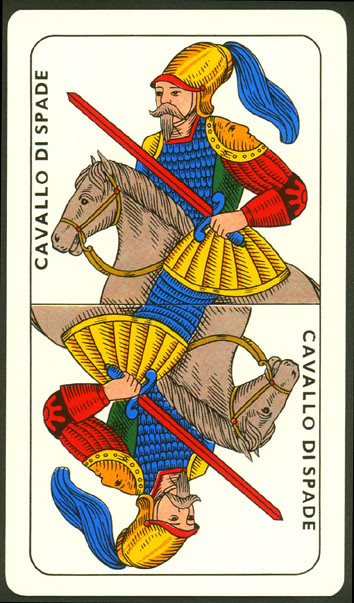This image is a scan of a tarot card or an unconventional playing card, distinctly lacking standard suits. The card, in Spanish, is labeled "Cavallo de Spade" (Knight of Swords). It portrays a man wielding a red and blue sword, mounted on a horse. The man is adorned in an old-fashioned Spanish infantry helmet with a blue tassel, blue chain mail, and a red coat accented with two golden shoulder pads. He has a light complexion, a beard, and a mustache. Notably, the card features a mirrored design, displaying the same image below the man's thigh, ensuring the image appears identical whether held upright or upside down. The card's background is completely white, and it rests on a dark green surface. The card’s artistic style suggests traditional hand-drawing with pencil, subsequently colored.